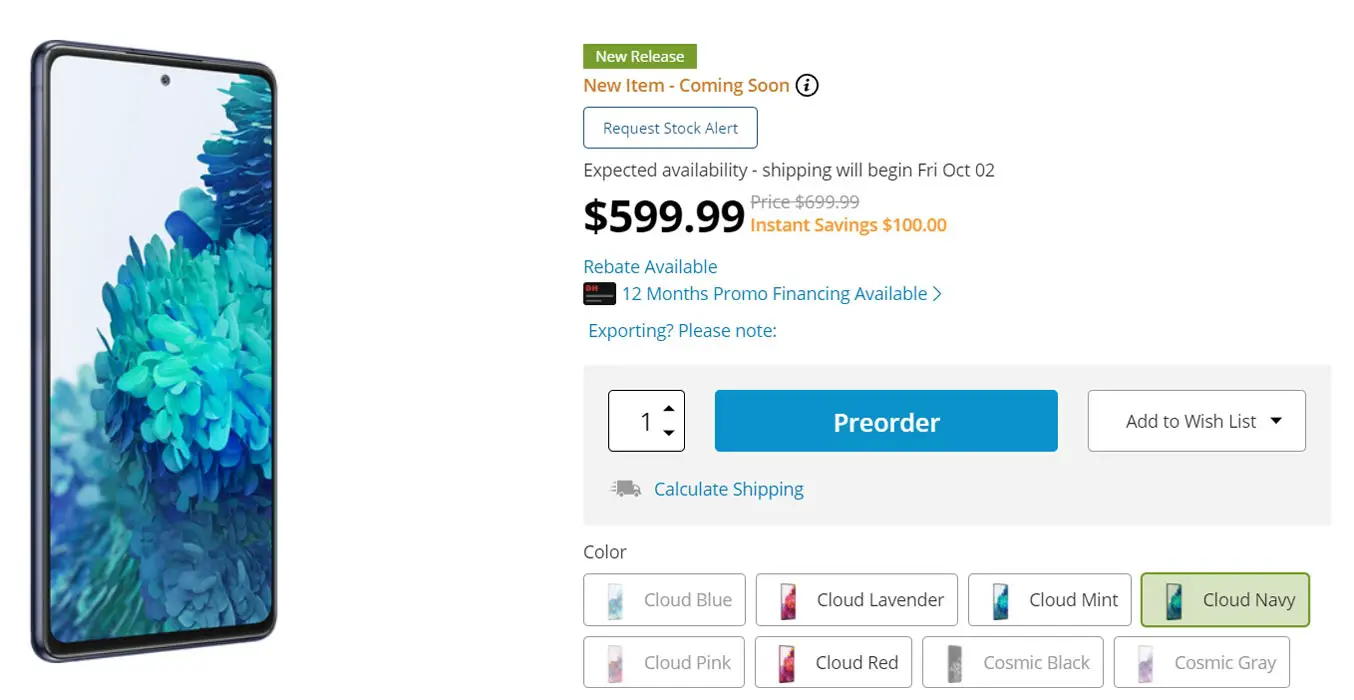A smartphone is prominently displayed on the left side of this image, showcasing a sleek design against a tranquil background. The image is part of an online store's product page. On the top right, a green banner with white text announces "New Releases." Beneath it, an orange label reads "New Item Coming Soon."

Immediately below, a blue button invites users to "Request Stock Alert." Following this, a detailed description reveals that the expected availability and shipping will begin on Friday, October 2, with the price set at $599.99 USD, discounted from $699.99, providing instant savings of $100 indicated in orange. 

Further down, blue text informs potential buyers of available rebates and a 12-month promotional financing option. A quantity selector shows one unit chosen. Adjacent to this is a prominent blue button inscribed with "Pre-order" in white text. To its right, a white button outlined in black offers the option to "Add to Wish List."

Additional blue text below allows users to "Calculate Shipping." The product is available in various colors, with "Cloud Navy" currently selected. Other color options include Cloud Blue, Cloud Lavender, Cloud Mint, Cloud Pink, Cloud Red, Cosmic Black, and Cosmic Grey. The diverse color palette is displayed on the bottom right of the page.